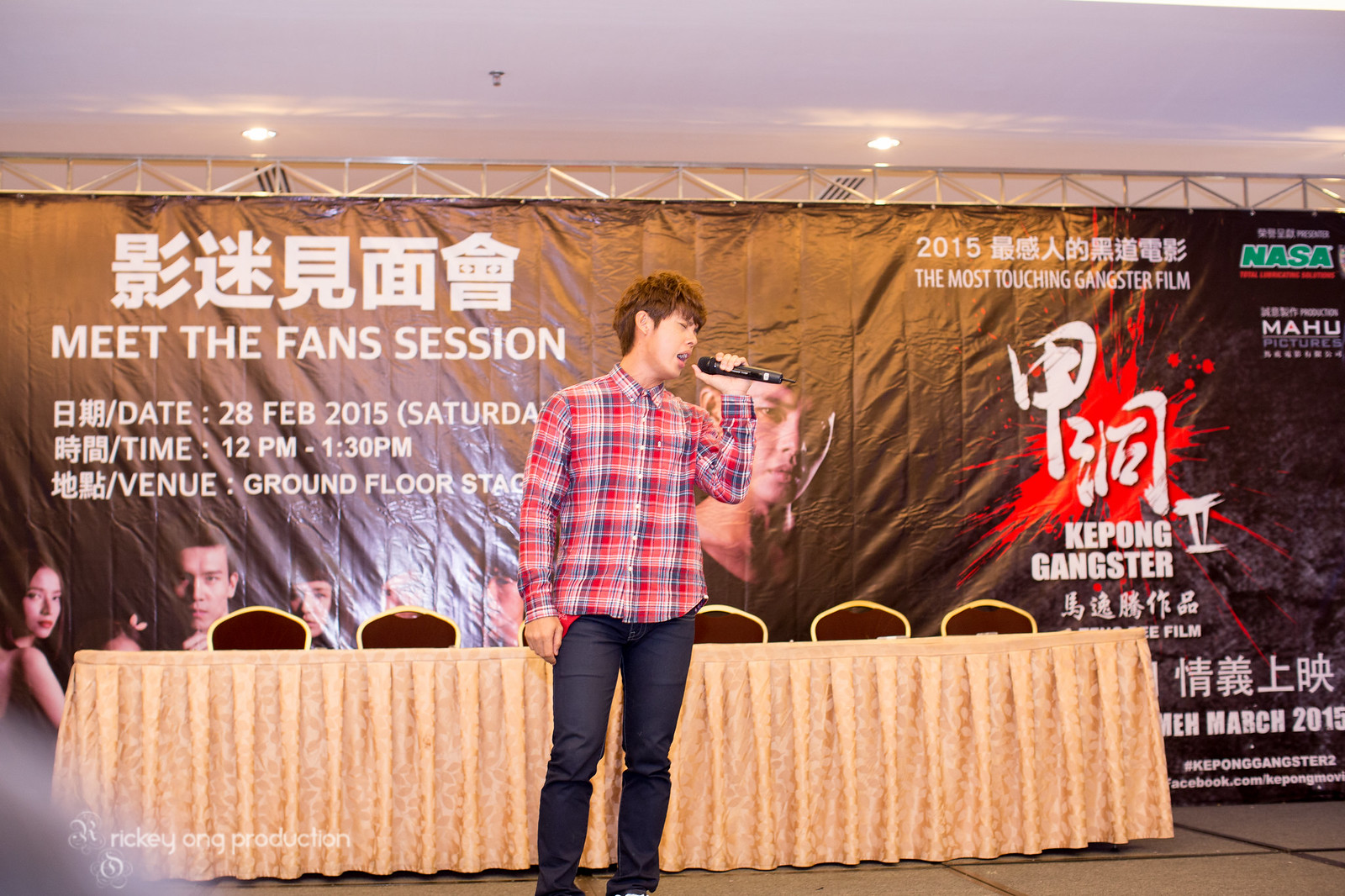This image features an Asian man in his 20s with long brown hair, enthusiastically singing into a microphone. He is dressed in a red and blue plaid shirt and dark blue jeans or black dress pants. Positioned in front of an orange curtain, the man stands before a table with six empty chairs, indicating a setting meant for a panel or forum. Behind him, a large black banner with both English and Asian script (Japanese or Korean) promotes a "Meet the Fans" session. The banner includes details in English: "28th February, 2015, Saturday, 12 p.m. to 1.30 p.m." on the ground floor stage. Prominently featured is the mention of "the most touching gangster film 2015, The Kibong Gangster," suggesting the man's association with, or fandom for, the film. Additionally, sponsorships such as NASA (likely not the space agency) and Mahou Pictures are visible on the banner.